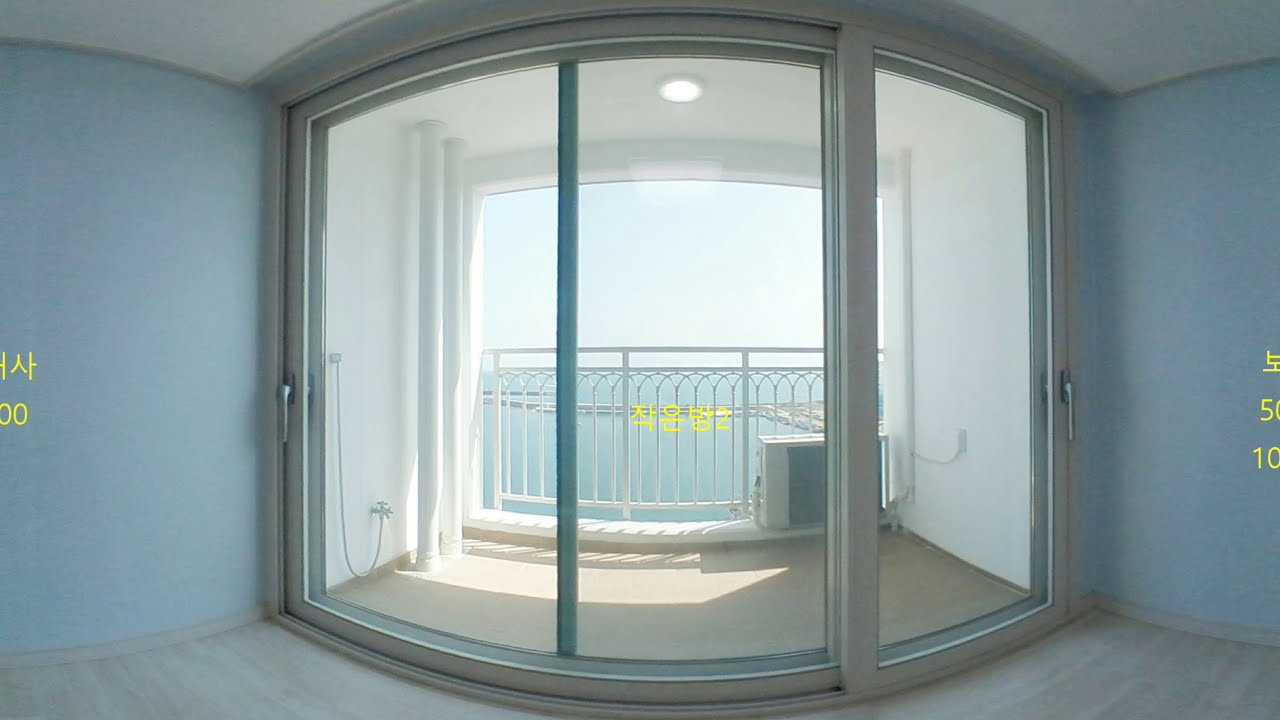This full-color photograph, horizontally rectangular without borders, captures an indoor scene on a sunny day. The image, likely taken in a room reminiscent of a hotel room or similar minimalistic space, features laminate gray flooring, tropical blue walls, and a white ceiling. Across the middle, yellow text in what appears to be an Asian language, possibly Korean, is presented centrally, as well as on the left and right sides of the image. Central to the composition is a large, rounded patio door with three panes, providing a view onto a small, enclosed balcony. The white-railed balcony, adorned with small pillars and a hose with a spigot on the left, offers a picturesque overlook of blue water, white clouds, and a bright sky. Additionally, there is an AC unit on the balcony and a small light, possibly white or red, that is turned on.